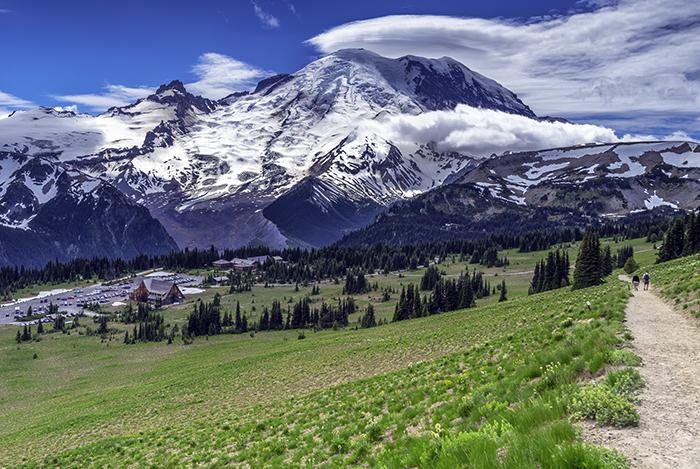This image captures a stunning daytime view of Mount Rainier with its snow-capped peaks standing majestically against a clear blue sky intermixed with scattered white clouds. Foreground details include a lush, grassy, hilly area with a verdant valley of tall pine trees. A dirt trail winds through the right side of the hill, and two hikers can be seen making their way up this path. To the left, there's a wooden building beside a parking lot filled with numerous cars, highlighting the accessibility and visitor-friendly nature of this location. The scene also features a small village setup with various huts and houses, underscoring the blend of natural beauty and human habitation. Overall, it's a picturesque snapshot of the iconic Mount Rainier and its surrounding landscape.